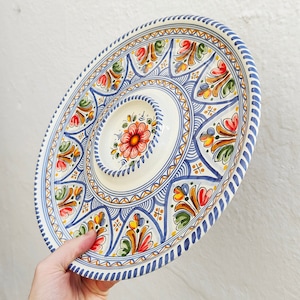The image features a ceramic decorative plate held by a white-skinned hand emerging from the lower left corner of the frame. The hand, appearing to be the left hand with its thumb facing left, is holding a circular plate characterized by intricate multicolored patterns. The plate has a white base with blue vertical lines forming a striped border around the edge. Just within this, there is a sequence of blue borders, and moving inward, a series of golden and blue round designs.

Further into the design, there are floral and geometric patterns with shades of orange, green, yellow, red, and blue. Notably, there are arch shapes with floral details, X shapes filled with yellow dots, and blue concentric circles, creating a visually rich tapestry. The centerpiece of the plate is an upraised circular section, slightly elevated, with a white background encircled by a blue border about an eighth of an inch high. This raised center features a vibrant red and yellow flower set against a predominantly orange field, adding a focal point to the elaborate design. The background of the overall image is a plain white-gray wall, providing a neutral backdrop that highlights the vivid colors and intricate patterns of the plate.